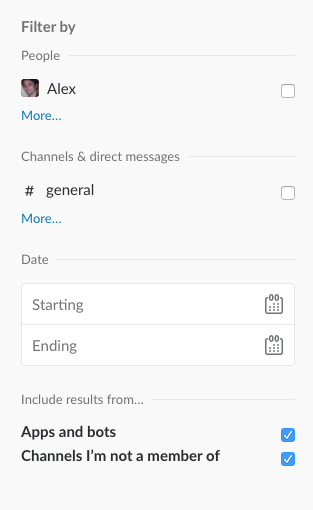This image is a detailed screenshot of a filtering interface on a cell phone.

At the top left corner, the words "Filter by" are displayed in bold black letters. Directly below that, aligned to the left, is the category "People" also in bold black letters, with a vertical line to the right separating it from other categories. Beneath "People," there is a small square thumbnail of a person who appears to be a man with dark hair and pale skin. Adjacent to the thumbnail is the name "Alex" in black text. On the far right, there is an empty white checkbox.

To the left of this section, the word "More" in blue with a set of three ellipses follows, indicating an expandable menu option.

Further down, the section title "Channels and direct messages" is printed in gray. To the left below this title is a hash symbol, followed by the word "General" in black letters. Again, to the right, there is an empty checkbox. A similar "More" option with blue text and three ellipses is present on the left under "General."

Continuing downwards, the next gray text category is "Date." Beneath this category, there are two horizontally aligned rectangles. The top rectangle includes the word "Starting" on the left and a calendar icon in gray on the right. The bottom rectangle contains the word "Ending" and another gray calendar icon to the right.

Further down, "Include results from" is displayed in gray, followed by three clickable ellipses. Below that, the bold black words "Apps and bots" appear on the left with a corresponding blue checkbox featuring a white checkmark on the right. Finally, at the very bottom, the phrase "Channels I'm not a member of" in bold black letters is situated on the left, accompanied by a blue checkbox with a white checkmark to its right.